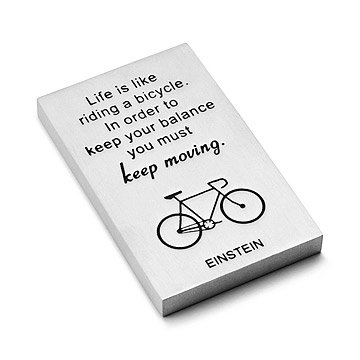The image features a canvas-like artwork, square in shape, with a slightly off-white background and black lettering. Positioned centrally and laying at a diagonal angle on a completely white surface, the artwork presents a motivational quote that reads, "Life is like riding a bicycle. In order to keep your balance, you must keep moving." The phrase "keep moving" is emphasized in bold cursive writing. Below the quote, there is a simple, black illustration of a ten-speed bicycle with handlebar hoops down. At the bottom, the word "Einstein" is written in black. The canvas edges, particularly on the left-hand side and bottom, are darker, suggesting shadow or a lack of light reflection. This elegant piece, suitable for wall hanging, combines inspirational text with minimalistic illustration, making it an ideal addition to any artistic display.